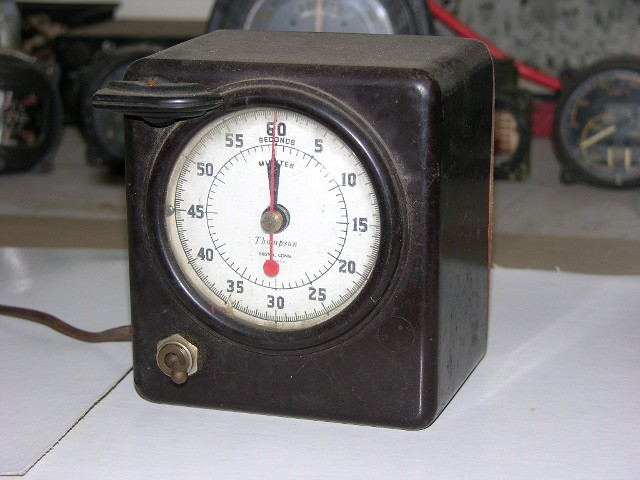The image portrays an old, dusty, square black box that suggests it might be a stopwatch or a countdown timer. The box exhibits slight rust, contributing to its vintage appearance. Positioned in the lower left-hand corner is a small copper dial that functions as a switch, allowing you to turn the device on and off. The face of the box is white and prominently displays the word "Thompson" in the center, accompanied by some other indistinct words. A gold knob is situated in the middle, with a red hand extending upwards towards the top, pointing to "60 seconds." Surrounding the face in a clockwise direction are numerals marking every 5-second interval, from 5 to 55, with each second denoted by individual tick marks. The box rests on a white table, with a background featuring wallpaper and a wheel visible in the distance.